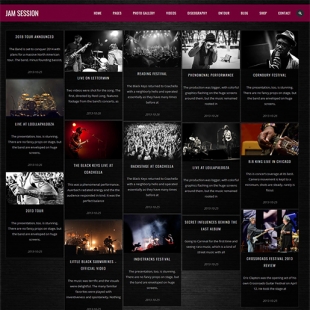The image depicts a nostalgically small snapshot reminiscent of mid-2000s websites, such as PureVolume. It likely advertises a 'jam session,' featuring several bands. The miniature visuals show performers on stage, silhouetted against a black background. A vibrant red menu bar crowns the website, enhancing the era-specific design. Though details are minimal due to the image size, silhouettes of enthusiastic crowds, musicians’ faces, and drum sets are discernible, evoking the raw energy of live performances.